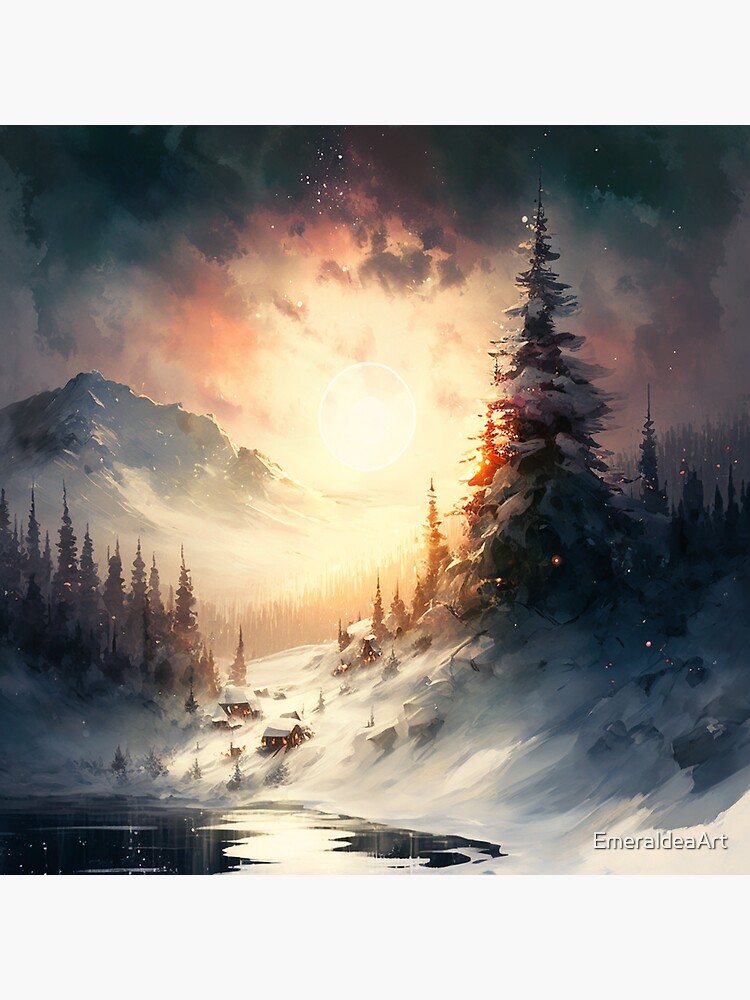This image, titled "Emerald Art," depicts a captivating winter scene, skillfully rendered to resemble an oil painting with possible computer-generated elements. The focal point of the artwork is a serene valley illuminated by a bright celestial body, which looks almost like a moon—shining prominently through a cloudy sky that ranges in hues from warm yellow to dark gray. The sky's illumination suggests a dawn or dusk setting, casting a calming, almost fantasy-like atmosphere.

In the foreground, a partially iced-over pond occupies the bottom left, its surface reflecting the glow from the sky. Above the pond, nestled on a snow-covered hillside, are three small brown wooden houses, their windows warmly lit, contrasting against the cold landscape. The roofs of these cozy cottages are blanketed with snow, adding to the serene winter ambiance.

To the right of the houses and partially surrounding them are majestic fir trees, heavily laden with snow, framing the scene with their dark, wintry presence. These evergreens continue to line the hillside, creating a natural border that enhances the depth of the painting.

Dominating the background is a grand snow-capped mountain, overseeing the tranquil valley below. This mountain is complemented by a range of smaller tree-covered hills, further enriching the scene with layers of natural beauty. The landscape captures the austere yet stunning essence of a Nordic winter, making it reminiscent of an idyllic Christmas card.

The bottom right corner of the image features a watermark in small white letters, identifying the artwork as "Emerald Art," underscoring the artistic craftsmanship behind this detailed and enchanting winter tableau.